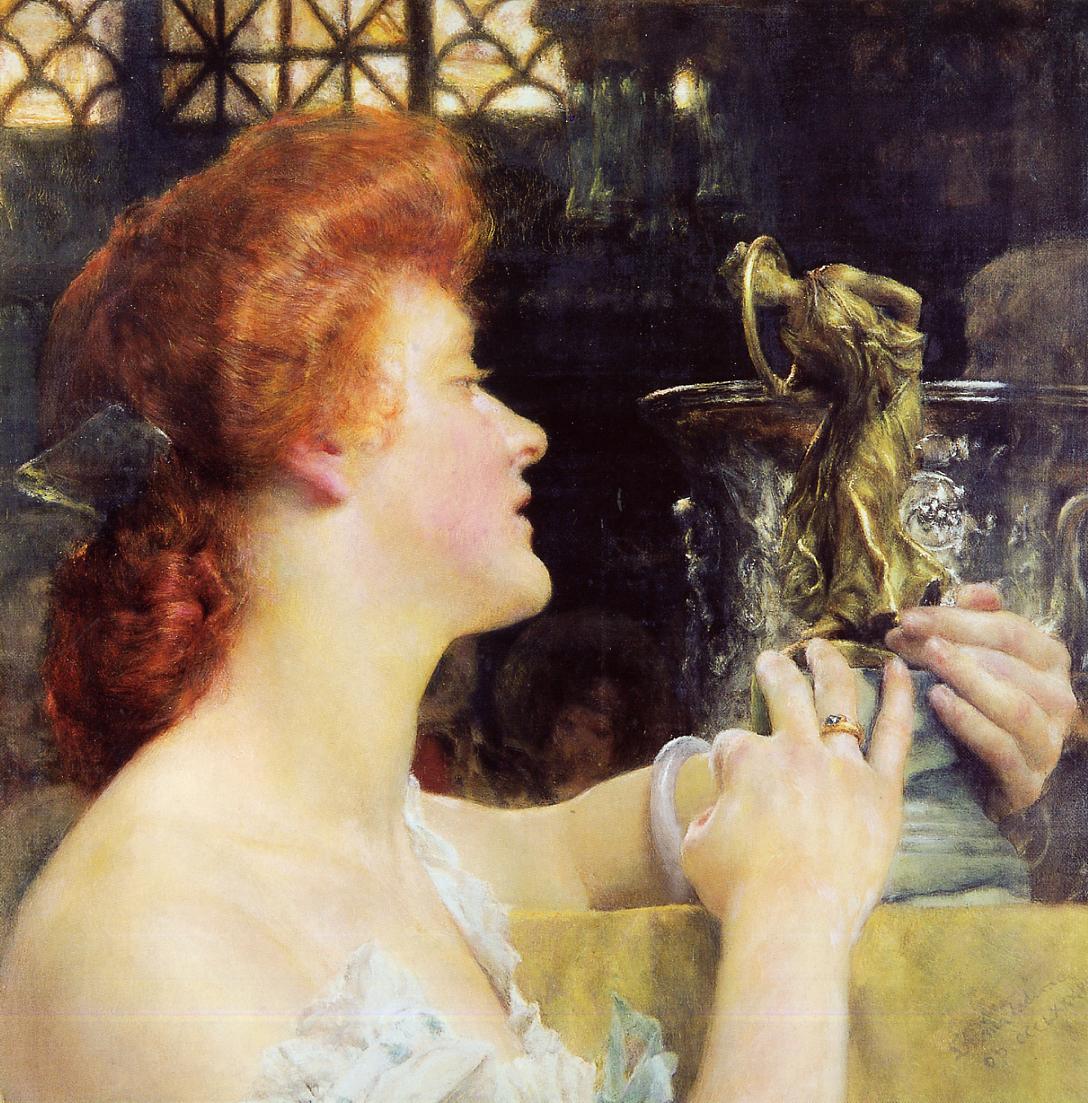In this detailed and lifelike painting, a red-haired woman with fair complexion is depicted sitting on a green couch. We see her from the shoulders up, with her long hair gathered at the nape of her neck with a clip. The woman is dressed in a white gown and is gazing admirably at a small bronze statue, which she cradles on a stone pedestal. The statue, depicting a woman bending over as if in pain, has her arms positioned behind her back, possibly bound, and features a large brass ring around her neck. The scene takes place in an interior room, evidenced by the detailed window with intricate, X-shaped panes and rainbow-shaped patterns, along with a silver vase placed adjacent to the statue.